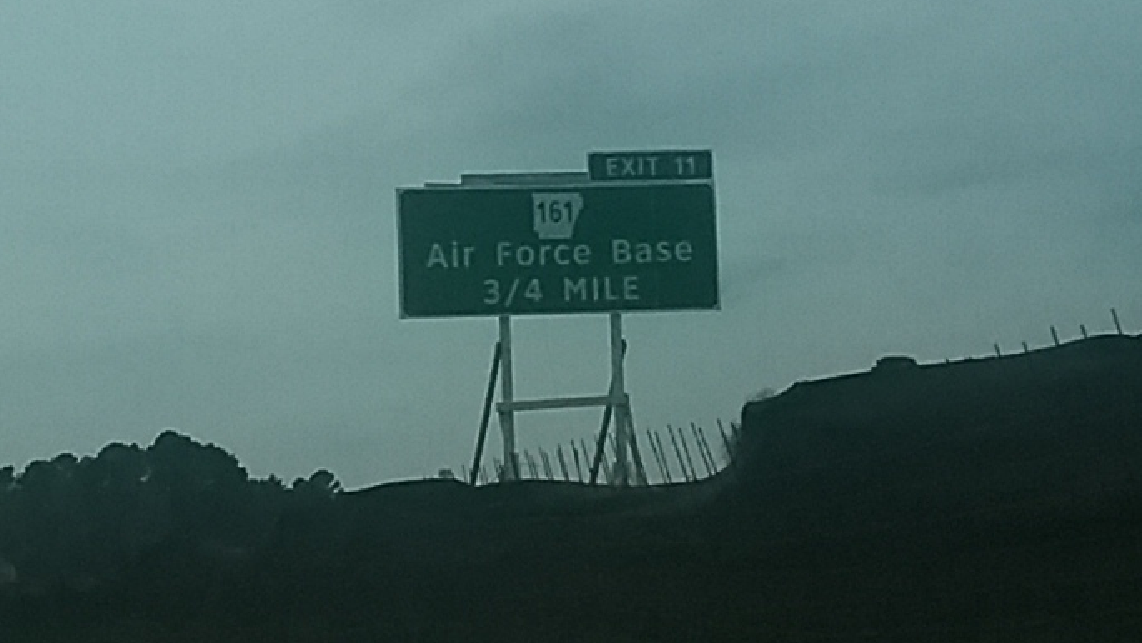On a cloudy day, a green road sign is prominently displayed in the center of the image, taken while driving. The sign, focused sharply, features a silhouette of the state with "161" inside it, depicted in white against the green background. Below this, in white letters, it reads "Air Force Base 3/4 mile," signaling the distance to the base. Above this is a smaller sign indicating "Exit 11." The signs appear to be mounted on a structure on a hillside, with fencing visible at its base, suggesting protective measures like razor wire. In the lower left corner of the photo, dark, indistinct foliage can be seen, probably trees along the roadside and hill.